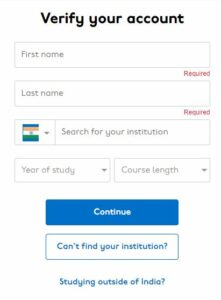The image depicts a verification page with a white background. The page's primary purpose is to verify user accounts, with a mostly black text layout. At the top, there's a bold black header stating "Verify Your Account." Below this header, there are input fields for "First Name," "Last Name," and "Search for Your Institution." The fields for "First Name" and "Last Name" have red text labeled "required" at their bottom right, indicating that these fields are mandatory and cannot be skipped.

Towards the bottom of the page, there's an Indian flag, displaying the colors saffron (mistakenly described as yellow), white, and green, alongside sections to specify the "Year of Study" and "Course Length." 

Two buttons are located near these sections: the first button is blue with white text reading "Continue," and the second is white with blue text that says "Can't find your institution?" which users can click if they're unable to locate their institution in the search.

Additionally, at the very bottom of the page, there's a blue text link which reads "Studying outside of India?" followed by the Indian flag.